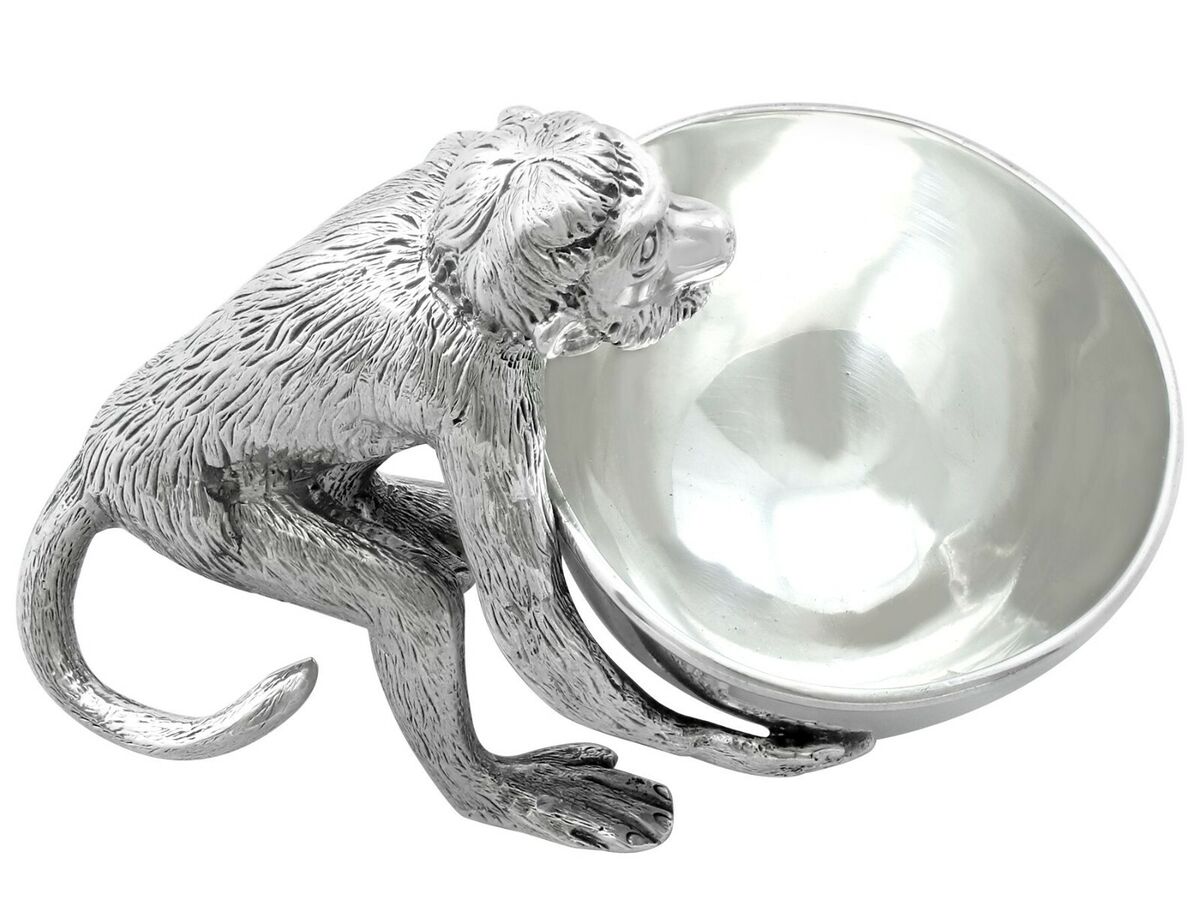Against a pristine white background stands a captivating silver sculpture depicting a monkey holding an opalescent, eye-like sphere. The finely crafted monkey, rendered entirely in shimmering silver, exhibits a small body with disproportionately long arms and legs, and a characteristically curled tail. Positioned to the left of the large, iridescent sphere, the monkey's right and left arms are extended beneath the spherical object, supporting its weight. The sphere itself is roughly the same size as the monkey and has an ethereal, opal-like quality that allows one to see what resembles an eye, complete with a pupil and iris, encased within. The monkey’s detailed features, including its contorted expression and toes touching the floor, convey the strain of lifting the heavy, enigmatic sphere, adding an emotive dimension to the artwork.